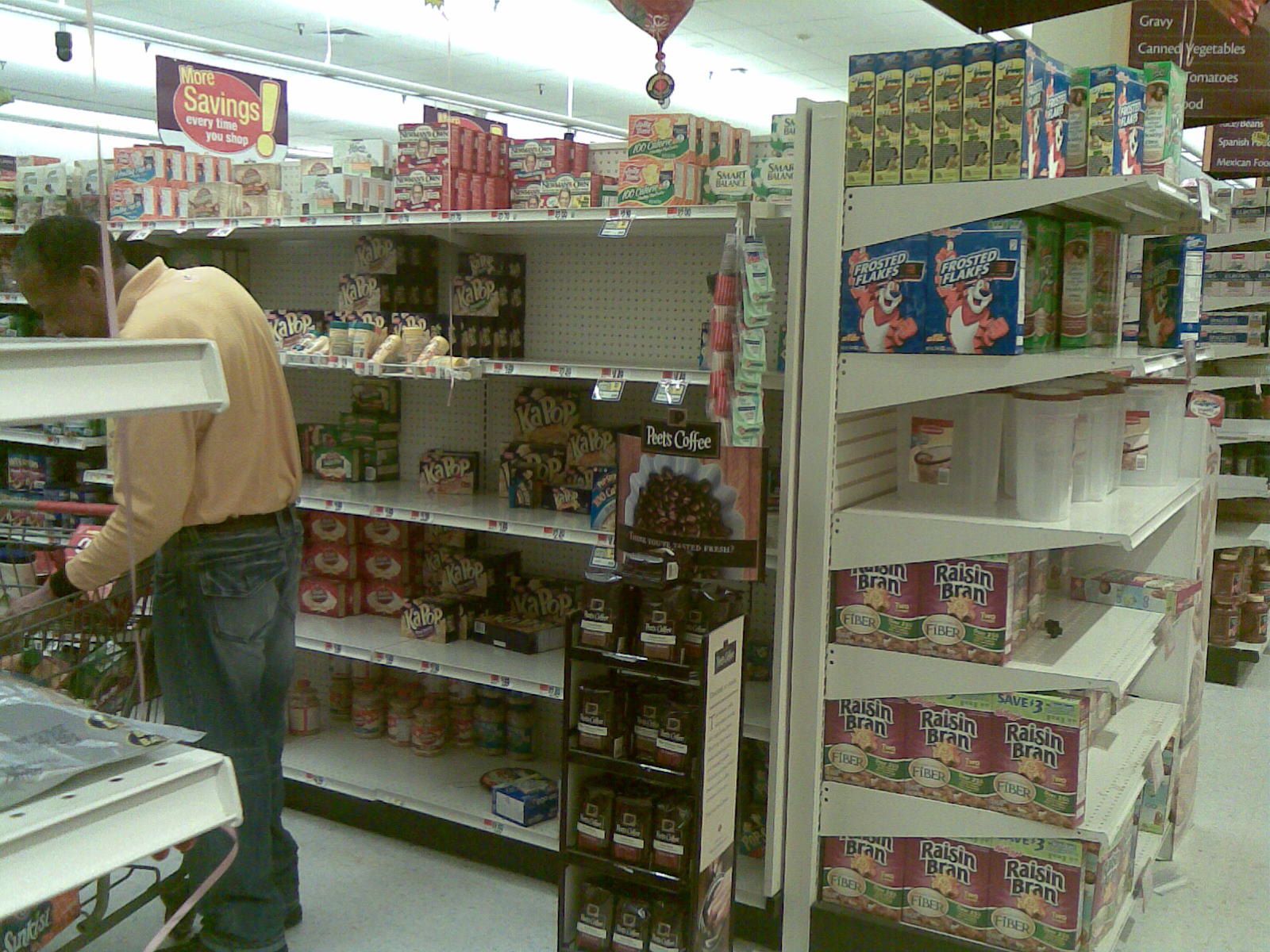The image captures a grocery store aisle featuring various food items prominently displayed on the shelves. In the foreground, a black man with black hair, dressed in a tan collared shirt and blue jeans with a brown belt, is browsing the aisle while pushing a shopping cart with a red handle. On the left side of the aisle, he faces white shelves that appear to be partially empty, with a small black shelf holding a few bottles of dark liquid. The aisle includes an end cap on the right showcasing Kellogg's Frosted Flakes in recognizable blue boxes with Tony the Tiger and Kellogg's Raisin Bran in purple boxes with white writing. There's also a stack of plastic gallon containers on one of the shelves. Additionally, the right side of the aisle features a variety of snack foods, including jars of Chiffy Pop on the bottom shelf and numerous types of microwave popcorn, such as Newman's Own. A stand for Pete's coffee is also visible, indicating the availability of coffee beans and potentially other products. The store is moderately lit, contributing to an overall somewhat dark ambiance, yet colorful due to the vibrant packaging of the products. A sign reading "More savings every time you shop" hangs above, reinforcing the typical grocery store environment.